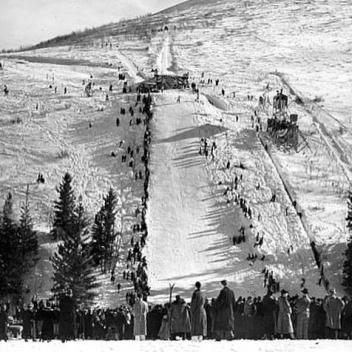This vintage black-and-white photograph captures a bustling winter scene that seems to be a historic skiing event from the 1950s. The image, vertically rectangular with no border, is taken from a higher vantage point, looking down on a snow-covered slope. The central feature is a smoothed-out ski run, indicating it is prepared for a skiing or sledding race. Spectators bundled up in long wool coats line both sides of the slope, forming a clear path for the skiers. At the bottom of the hill, a throng of onlookers gathers, their attention focused upward. Amidst the crowd on the slope, one skier can be seen making their descent. A platform constructed from metal or wood, possibly for judges, is visible alongside the slope. Sparse trees dot the landscape, and a tent or some structure appears in the background, hinting at event facilities. The photograph exudes a sense of nostalgic charm, reflecting a historical moment for a town or perhaps a notable skiing competition.